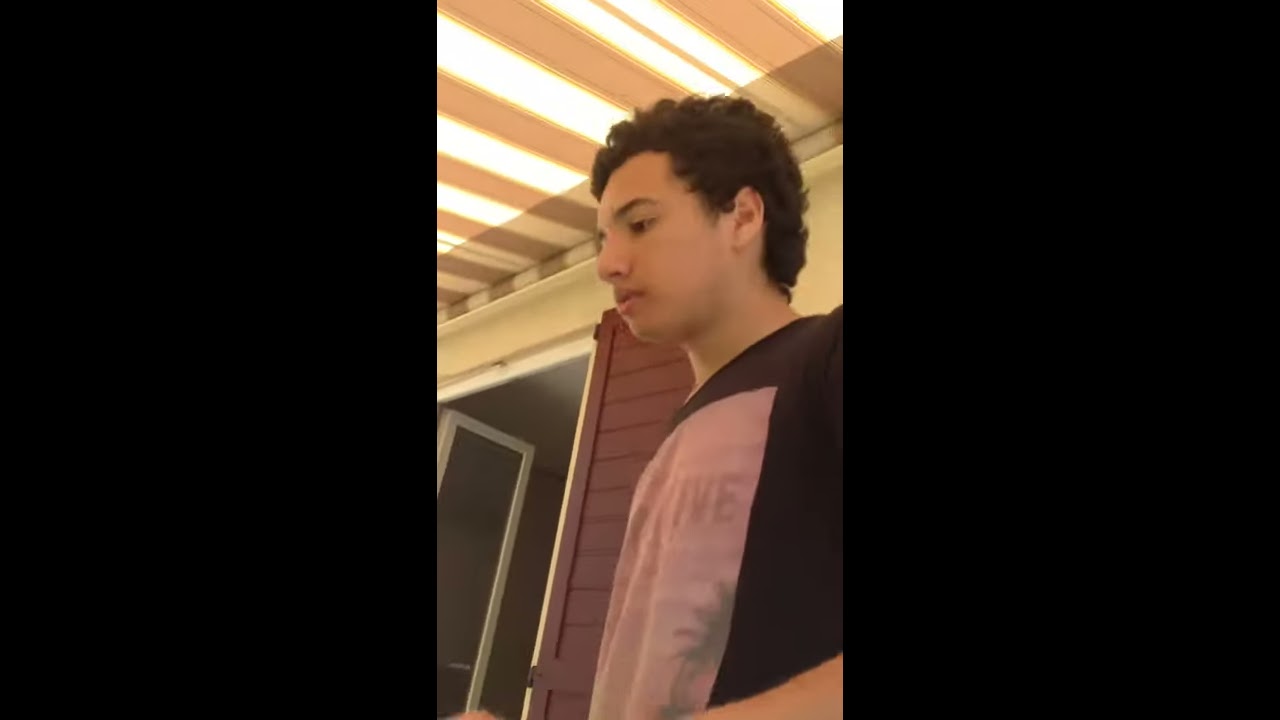This image features a central photograph flanked by wide, solid black panels on either side. The photograph depicts a young man with short, dark curly hair, presenting as male and displaying a profile view, looking slightly downward towards the viewer's left. He has lighter skin with a touch of a tan and dark black eyebrows. He is wearing a black short-sleeved t-shirt that has a design featuring a square, possibly with the word "live" printed on it. 

The young man stands in front of what appears to be a house or perhaps a trailer. Behind him, a brown shutter is visible alongside a white-framed door, through which an interior wall is partially seen. Above him, a beige border and an awning with white and beige stripes add detail to the scene. The awning suggests that sunlight is being filtered, casting subtle glare and indicating an outdoor setting.